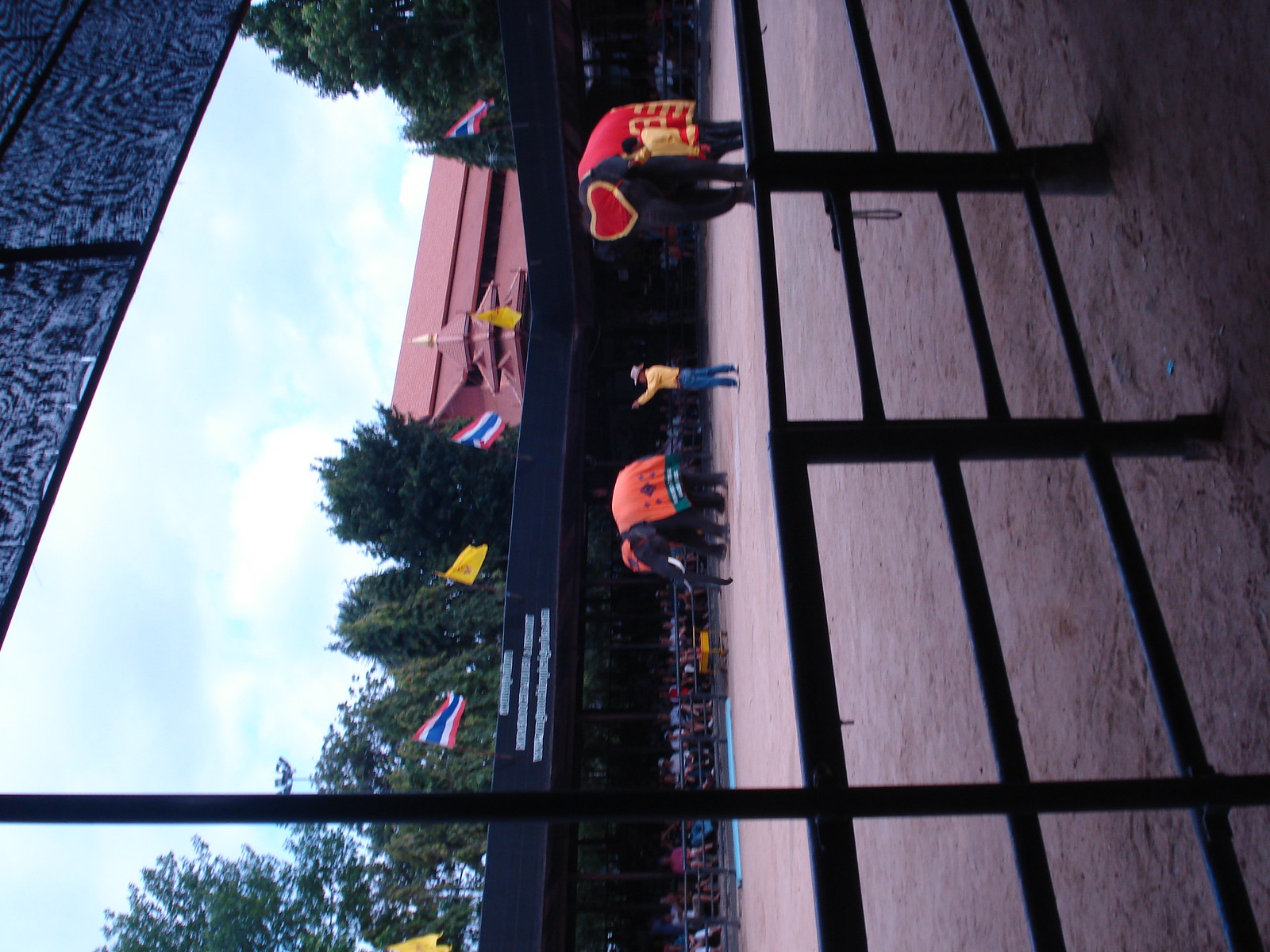This color photograph, rotated 90 degrees to the left, depicts a vibrant scene in an open-air coliseum or courtyard. The image is viewed through a dark metal gate with three horizontal bars and a latch. The ground on the right side of the image is beige and earthen, while trees stretch skyward on the left. 

In the middle, two dark-colored elephants are adorned with ornate coverings; the elephant on the right wears a red vest with gold stripes and a red headpiece bordered in gold shaped like a heart, while the elephant on the left sports an orange and green vest with a matching headpiece. Both elephants have visible tusks. 

Leading the elephants are two trainers. The trainer on the left is clad in a yellow long-sleeved shirt, blue jeans, and a light-colored hat, and the trainer on the right wears a yellow shirt with dark pants. 

In the background, a grandstand filled with spectators is visible, suggesting a circus or public event. The grandstand is topped with alternating Mexican national flags and yellow flags, and beyond are tall green trees and a reddish-roofed structure with a steeple. The sky above is light blue with patches of clouds.